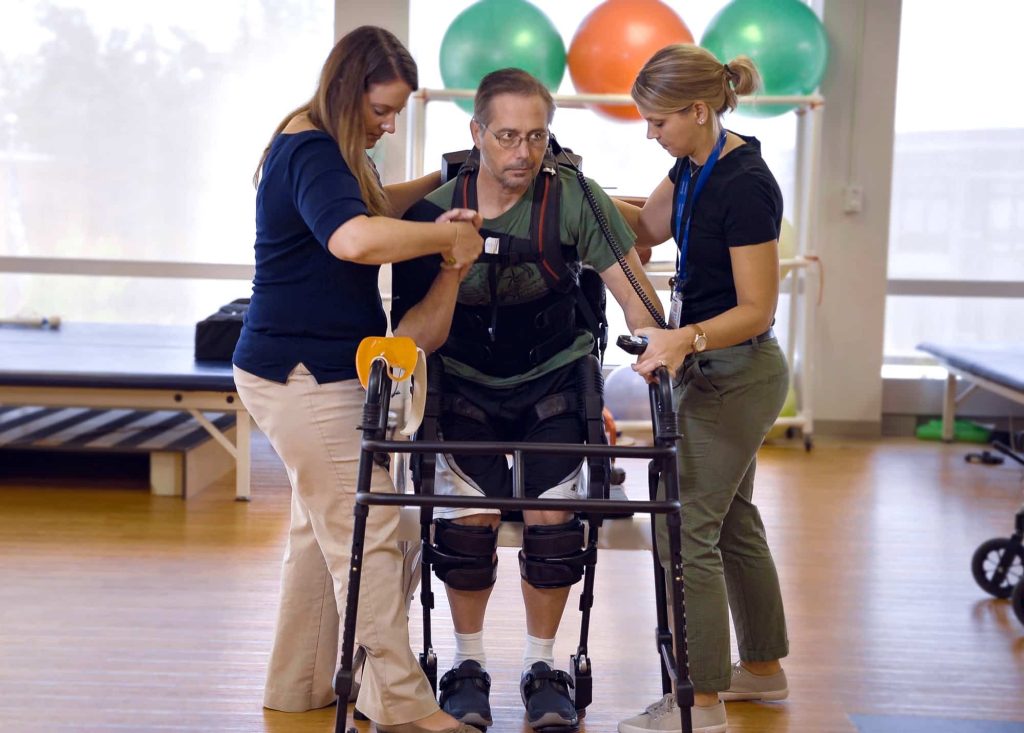The image depicts a middle-aged man undergoing physical therapy in an indoor setting, likely to aid his mobility. The man, who has short, graying hair, a grey beard, glasses, and a five o'clock shadow, is using a black brace-type walker. He is wearing extensive braces that are strapped to his shoes, knees, and up around his shoulders, along with additional padding and straps that go around his neck and crotch, possibly connected to a remote control for movement stimulation. On either side of him, two female physical therapists are assisting him; the therapist on the right wears a short-sleeved black t-shirt, army green pants, and flat sneakers with her hair pulled up, while the therapist on the left is dressed in a dark blue t-shirt and white pants. Observing him with meticulous attention, they are aiding in his recovery process. The room has wooden flooring, and in the background, there are windows, benches, and a rack with several large exercise balls – the most prominent being an orange ball flanked by two green ones.